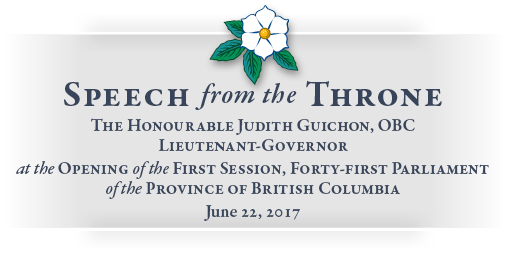The image is a digital notice or card featuring a white background and a horizontally oriented, light gray rectangular shape that fades to white on both ends. At the top, there is a simple design of a white flower with petals radiating from a yellow center, accompanied by four green leaves at the base. The text on the gray ribbon is in a serif font and predominantly in all caps, except for minor prepositions. The main heading reads, "Speech from the Throne." Below this, it states, "The Honorable Judith Guichon, OBC, Lieutenant Governor," followed by "At the Opening of the First Session, 41st Parliament of the Province of British Columbia." The date, "June 22, 2017," is positioned at the bottom of the text block. The overall feel is light and formal, with a gradient background supporting the presentation.